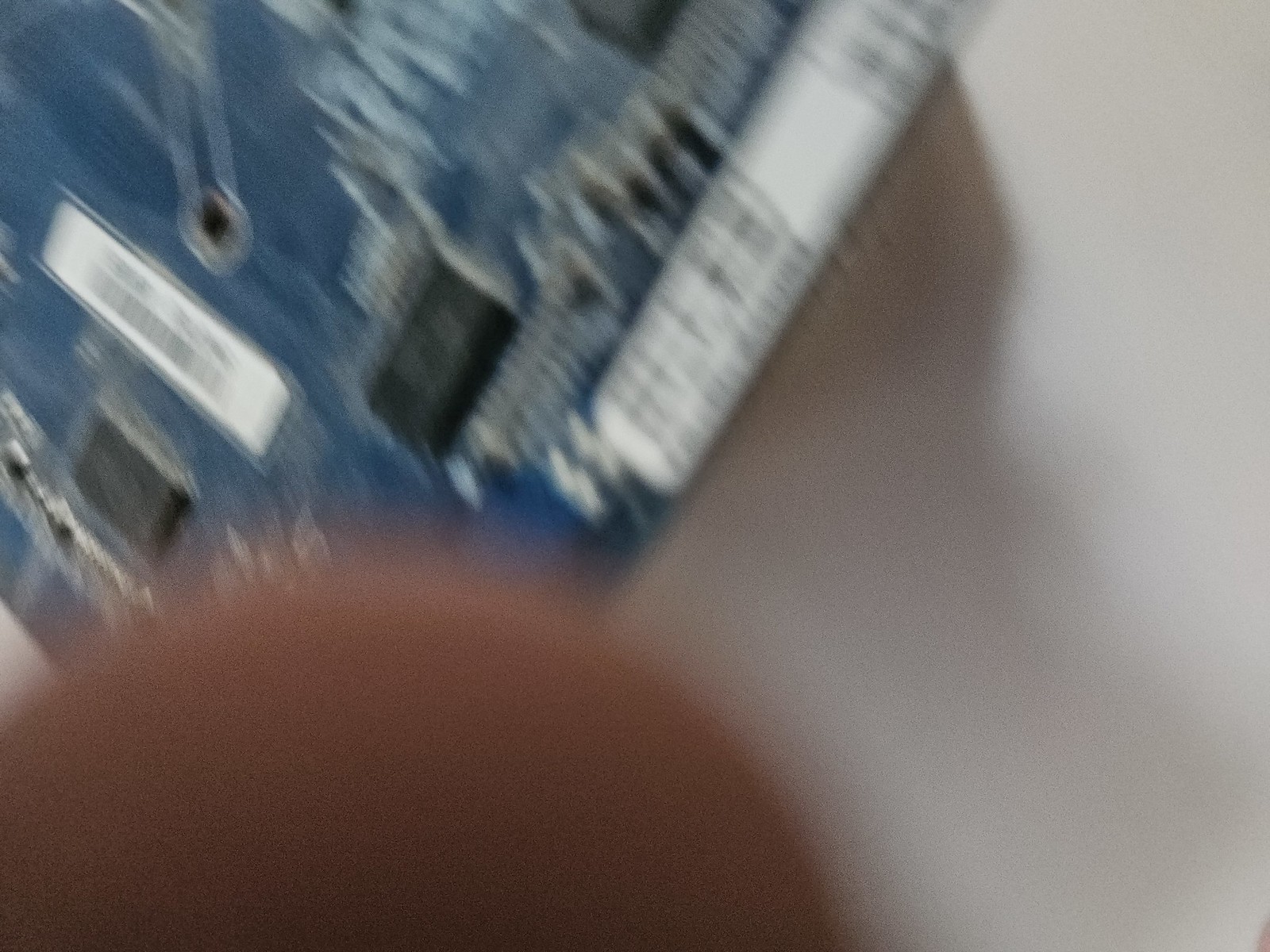The image depicts a highly blurred scene featuring two primary objects against a light gray wall with a shadow. At the bottom center of the image, there is a partially visible, faded circular shape with a brownish-purple hue, possibly the top half of an object. Above this, slightly off-center to the right, is a blue card-like shape with a white border. This object features two small black buttons and a rectangular white label. A series of white or light gray lines run through the design of the blue card. In the center of the card, there is a black hole encircled by a white outline. The right portion of the image is dominated by a light gray wall casting a shadow, adding to the overall obscure and indistinct quality of the scene.